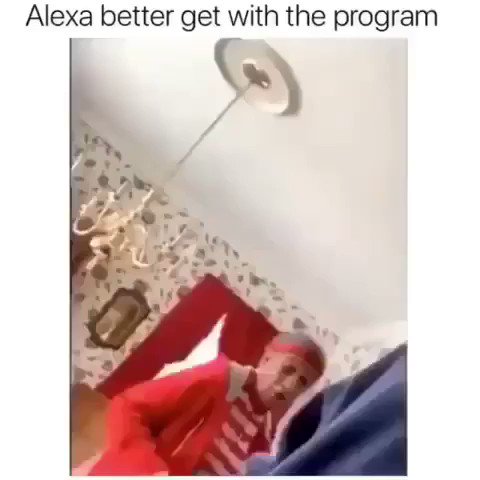The image depicts the interior of a room from a slightly tilted and blurry angle, approximately 35 to 45 degrees to the right. Dominating the center of the image is an elderly woman dressed in a red and white striped shirt, complemented by a red raincoat and a red headband. Her hair, lipstick, and accessories also embrace shades of red. Hanging from the white-painted ceiling is a chandelier, adding a decorative touch to the room. The background features intricately designed wallpaper, alongside a mirror. To the right of the mirror, a window adorned with bright red curtains frames part of the wall. In the vicinity of the woman's right side, there's a dark object, possibly black cloth or another person in a blue jacket positioned near the camera. The words "Alexa better get with the program" are inscribed at the top of the image in black. The overall scene is slightly skewed, rendering the elements at an angle.